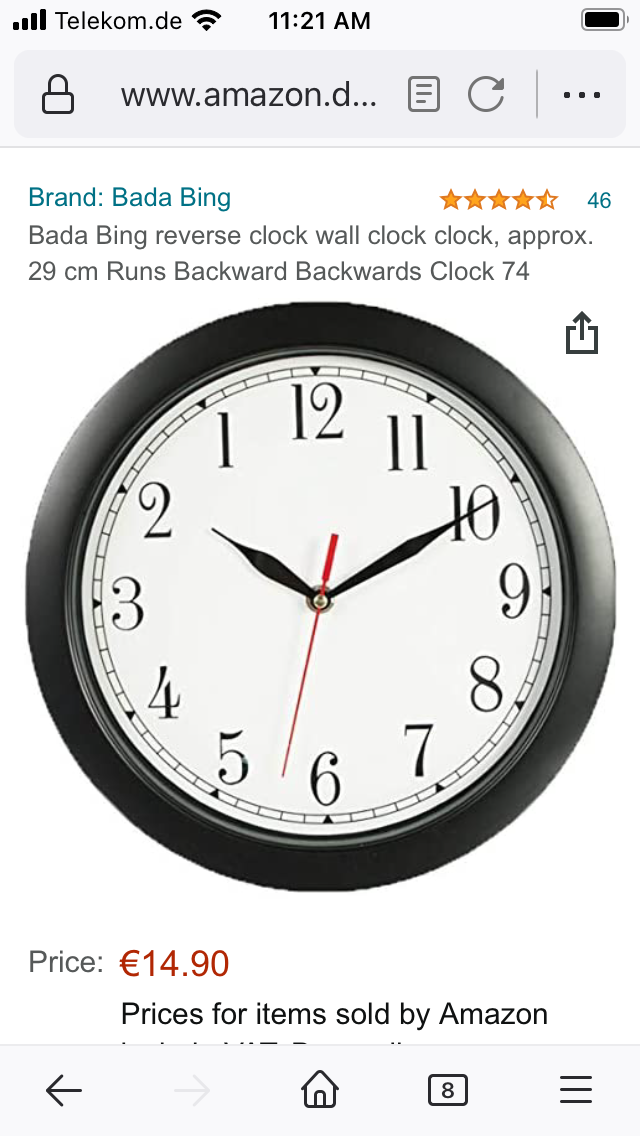The image displays a black, circular Brandering wall clock advertised on Amazon for €14.90. This unique clock features a white face with black numerals arranged in reverse order, and it runs backwards, presenting a quirky twist on a classic design. The clock, approximately 29 centimeters in diameter, has received high ratings—4.5 stars from 46 reviews. The hands are black, except for the red minute hand. The time on the clock is shown as 2:50, though due to its reverse mechanism, the numbers ascend counterclockwise with 12 at the top, 1 to the left, and so forth, with 6 at the bottom. The image seems to be taken from a phone screen that also shows a full battery, the time of 11:21 am, and a strong Wi-Fi signal.